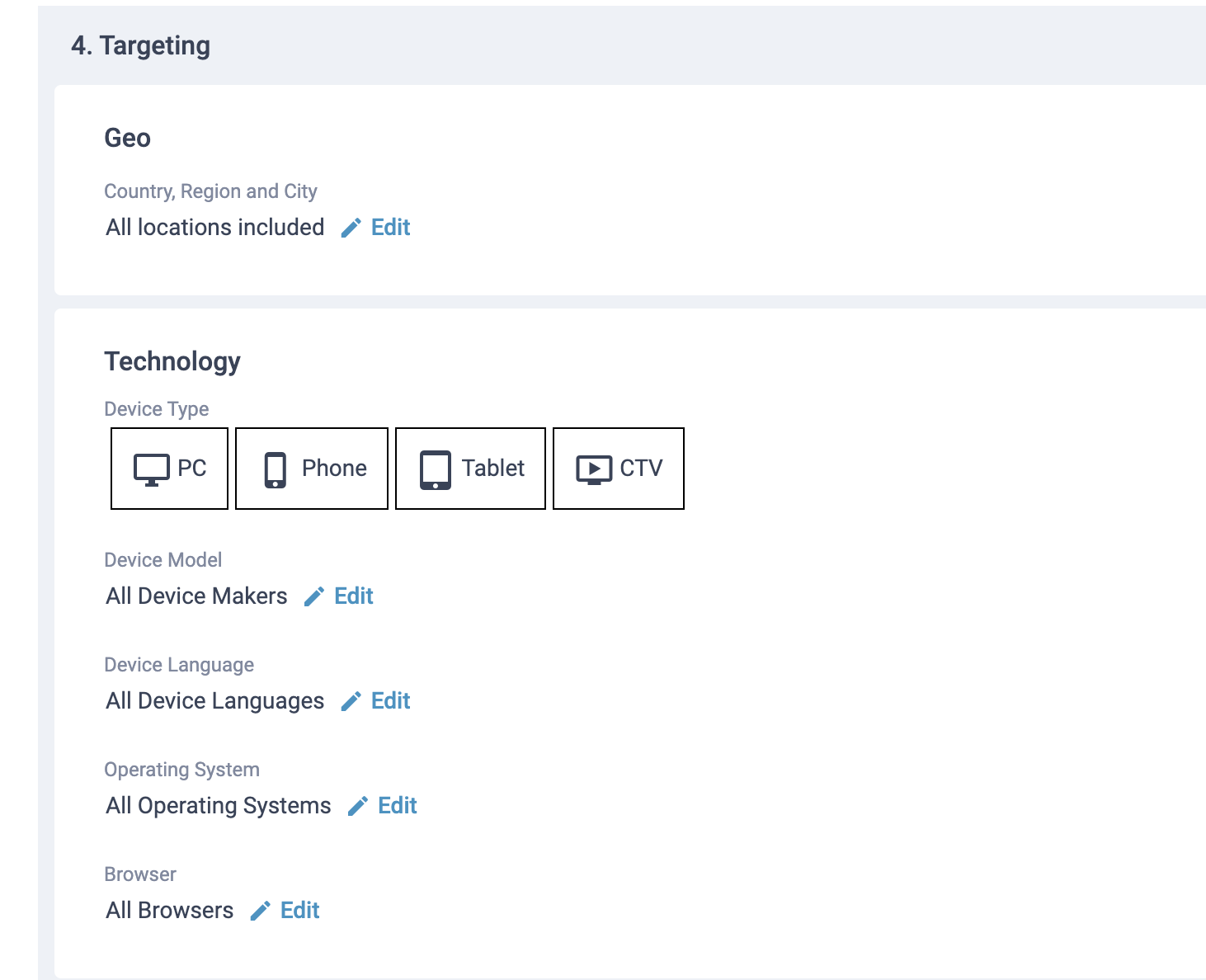Screenshot of a tablet displaying a setup page against a white background, primarily text-based. The top section features a narrow, pale blue banner with a heading on the upper left that reads "4. Targeting." Below, a white background with a subtle pale blue border lining the left side leads into the content. The first section is labeled "Geo" in dark blue print, with smaller text listing "Country, Region, and City." The current setting is "All locations included," accompanied by an editable icon and the word "Edit" in a lighter blue.

Further down, another white section is labeled "Technology" in the upper left corner. This section includes rows labeled "Device Type" displaying four selectable options—PC, phone, tablet, and CTV—with small corresponding icons. Below, "Device Model" is set to "All device makers," with an edit icon and link. Additional settings include "Device Language" displaying "All device languages" with an option to edit, "Operating System" set to "All operating systems," and "Browser" displaying "All browsers." This setup page appears to be before any configurations have been made.